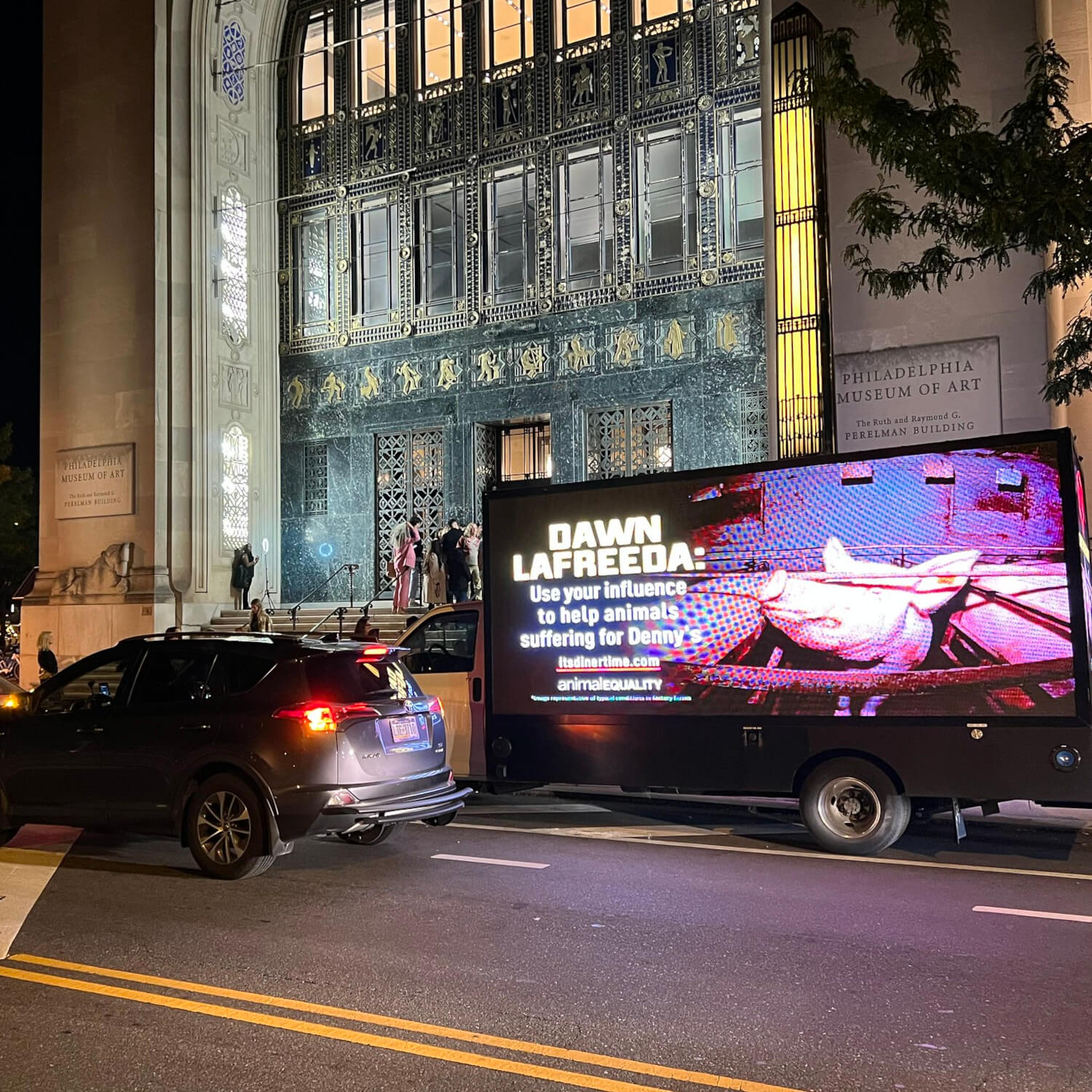This image depicts a night-time city scene in front of the Philadelphia Museum of Art, specifically the Ruth and Raymond G. Perelman Building. Dominating the foreground is a truck with a large electronic billboard attached, displaying a vivid and emotionally-charged ad. The ad appeals to Don LaFrida, urging him to use his influence to help animals suffering due to practices at Denny's, and features the URL "itsdinnertime.com" alongside the logo of the animal rights organization "Animal Equality". The advertisement is accompanied by a distressing image of a pig in a slaughterhouse, its eyes wide with fear. The museum's imposing, stone-clad façade with a grand archway and multiple windows serves as the backdrop. The entrance, marked by green marble and gold ornamentation, is lit up, and several people dressed for an event are visible near the doorway. A black SUV and a Honda CR-V can be seen navigating the city street, which is bustling with activity. The visual contrast between the moving vehicles and the static, striking billboard highlights a moment of intersection between urban life and advocacy.